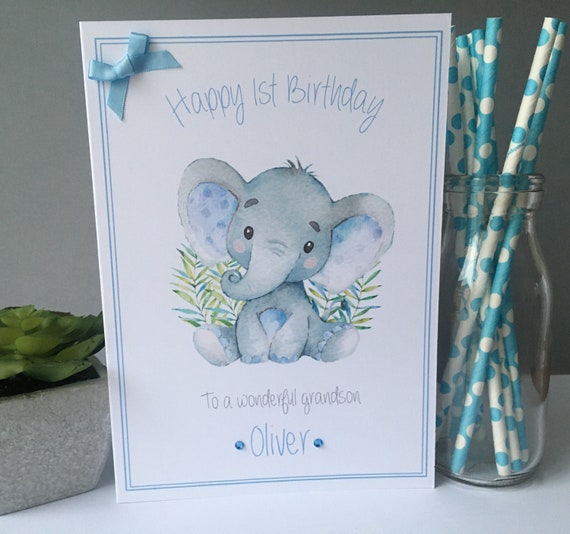The photograph showcases a meticulously arranged birthday card set against a white counter and wall. To the left of the card, a squat succulent thrives in a grayish stone planter, while on the right, a glass jar fashioned from an old-style milk bottle holds an assortment of paper straws adorned with electric blue and white polka dots. The focal point, a greeting card, features a pristine white background accentuated by a delicate blue double-lined border and a charming blue bow in the upper left corner. The card warmly wishes "Happy First Birthday" in a light, cursive-like font. Below, an adorable baby elephant, detailed with pink cheeks, blue accents on its ears and belly, and tiny blue toes, sits upright with a tuft of hair on its head, surrounded by subtle green and yellow foliage. The heartfelt message "To a Wonderful Grandson" appears in gray, followed by the name "Oliver" in blue, flanked by small blue stones.